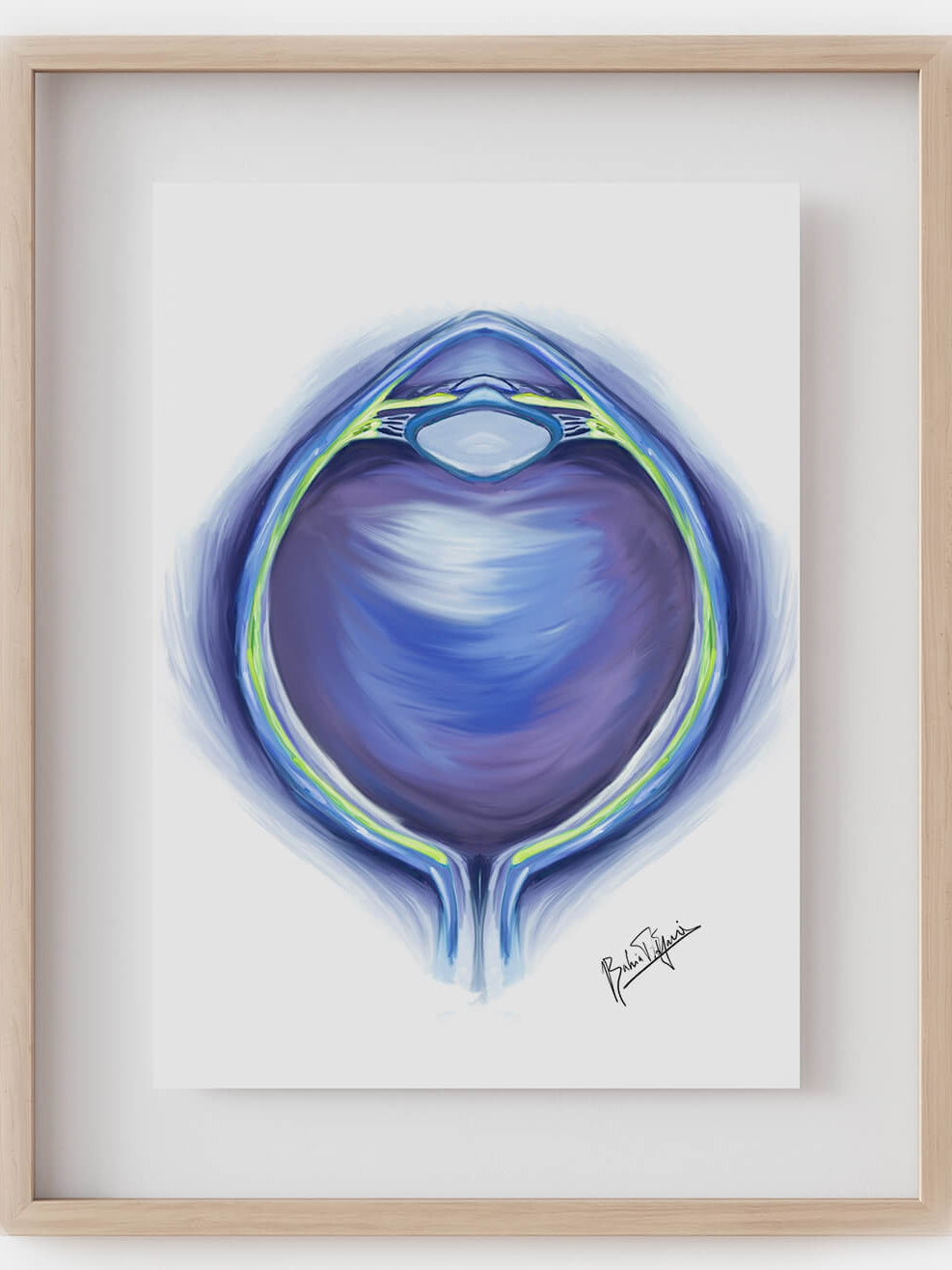The image depicts a framed painting set against a white background. The wooden frame is brown and rectangular, encasing a canvas that is predominantly white and slightly grayish. Central to the painting is an orb-like object resembling a cross-section of an eye, viewed from the top. This object is richly detailed with shades of blue and purple, highlighted by streaks of yellow and green lines encircling it. The eye-like shape also has a window-like feature with a lighter blue frame. At the bottom right corner of the canvas, there is a black, slanted signature that appears to read "Bahia Fadjura," though it is somewhat illegible. The entire composition gives the impression of a mix between anatomical art and a fantastical spacecraft, enveloped in a soft, ethereal glow.